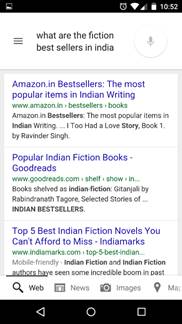This image, captured from a cell phone screen, features a digital interface dominated by a predominantly white background. At the top of the screen, a slim black rectangle contains three horizontal black bars next to the text "What are the fiction bestsellers in India?" and features a microphone icon for voice input.

The bottom of the screen is occupied by a thicker black rectangle, which houses three white icons: a triangle on the left, a circle in the middle, and a square on the right, reminiscent of typical navigation buttons.

Beneath the search query, three clickable options are presented. The first option, partially cut off at the bottom, displays in blue text "Amazon InBuilders," followed by "the most popular items in Indian writing" and a green clickable link labeled "www.amazon.in bestsellers in books." 

The middle option, also in blue text, reads "popular Indian fiction books — Goodreads" and includes a link to "www.goodreads.com" with the words "Shelf, show in" highlighted in green.

The final option references "Top five best Indian fiction novels" with the phrase "You can't afford to miss Indian marks" partially visible.

Each of these selections offers a different resource for discovering popular Indian fiction books.